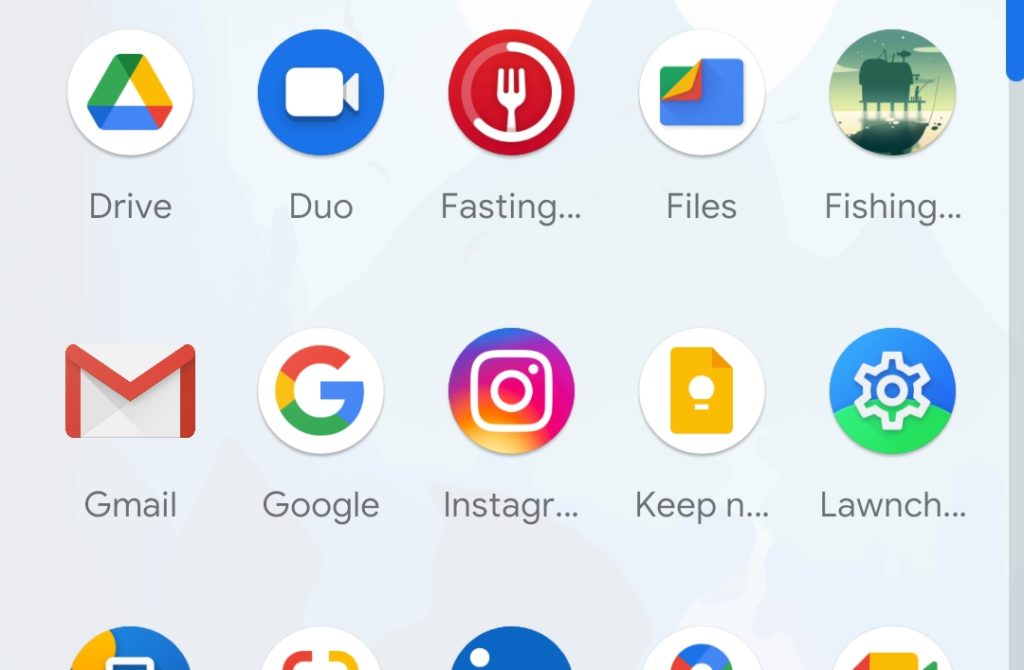This screenshot displays a variety of app icons neatly organized on a cell phone screen. Starting from the upper left corner and moving to the right, the first row of apps includes:

1. **Google Drive**: Represented by a distinctive triangle icon with three differently colored sides - green, yellow, and blue.
2. **Google Duo**: Recognizable by its blue circular icon featuring a white camera in the center.
3. **Fasting**: Marked by a red circular icon with a white circle inside it, which further encloses a white fork.
4. **Files by Google**: Illustrated by a blue rectangular icon. Inside, there is a green card within a pocket, topped with folded layers colored yellow and red in the top left corner.
5. **Phishing**: This icon depicts a potentially ambiguous image of a pier, showing what could either be a distant carnival or an oil rig.

On the second row, from left to right, the apps shown are:

1. **Gmail**: Featuring its simple yet iconic red and white envelope logo.
2. **Google**: Known by its striking 'G' logo in blue, red, yellow, and green.
3. **Instagram**: Displaying its recognizable gradient square with a white outline of a camera.
4. **Google Keep Notes**: Identified by its yellow lightbulb icon representing note-taking.
5. **Launch**: Spelled “L-A-W-N-C-H,” though the visual description of this icon is not included.

Unfortunately, the third row only shows the tops of additional app icons, which are not fully visible and thus their names or functions cannot be identified from this screenshot.